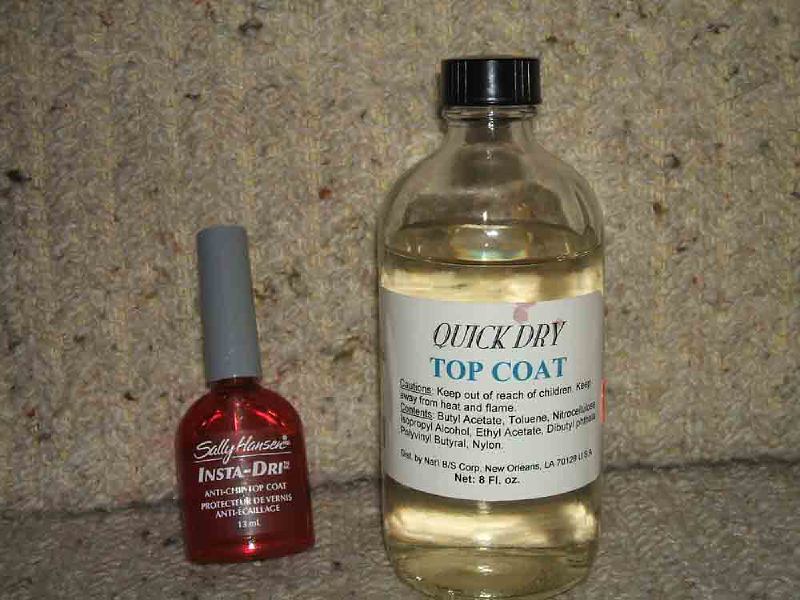The photograph displays two nail polish bottles positioned on a light brown, speckled fabric that appears to be a close-up of a couch or chair cushion with vertical stripes and scattered black and brown specks. The foreground shows these bottles slightly leaning back against the cushion. On the left is a small red bottle with a long gray cap, clearly labeled as "Sally Hansen Insta-Dry Anti-Chip Top Coat." The label also mentions protection features, though some text is obscured by glare. To the right is a significantly larger clear bottle filled with a transparent liquid, featuring a black screw-on lid. Its white label prominently reads "Quick Dry" in black text, followed by "Top Coat" in blue, along with cautionary details and ingredient information in smaller black letters. The larger bottle extends almost to the top of the image frame, emphasizing its size compared to the smaller bottle.